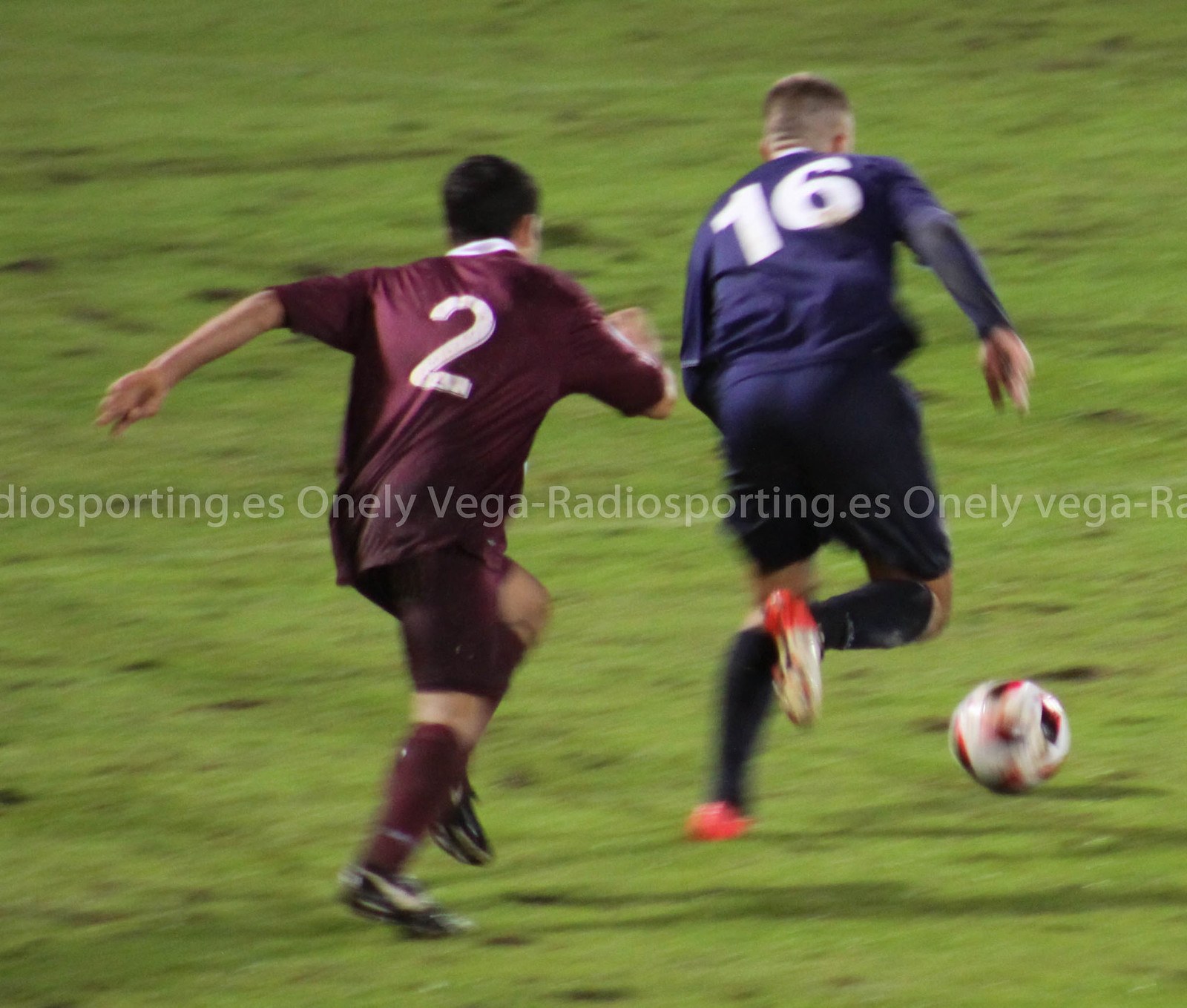This photograph captures an intense moment in an outdoor soccer game, viewed from behind. The image, slightly wider than tall, shows two men chasing a soccer ball across a green field, which appears blurry, emphasizing the action's speed. Both players are heading from left to right at a slight upward angle. The ball, located on the right side of the picture, is white with blue and red designs.

The player closest to the ball appears to be Caucasian with pale skin and a buzzed haircut. He is dressed in a navy, possibly bluish-purple, long-sleeved shirt featuring a white number 16 on the back, matched with shorts and knee-high black socks. His orange and white soccer cleats are visible as his knee lifts, poised to kick the ball.

Chasing him is a slightly shorter player with tanned skin and short black hair, clad in a maroon-colored uniform marked with a white number 2 on the back. He wears matching maroon socks and black and white cleats. With arms swinging in determination, he strives to close the distance.

A horizontal inscription, "onlyvega-radiosporting.es," repeats across the blurry green field, adding to the dynamic feel of this high-energy game moment.